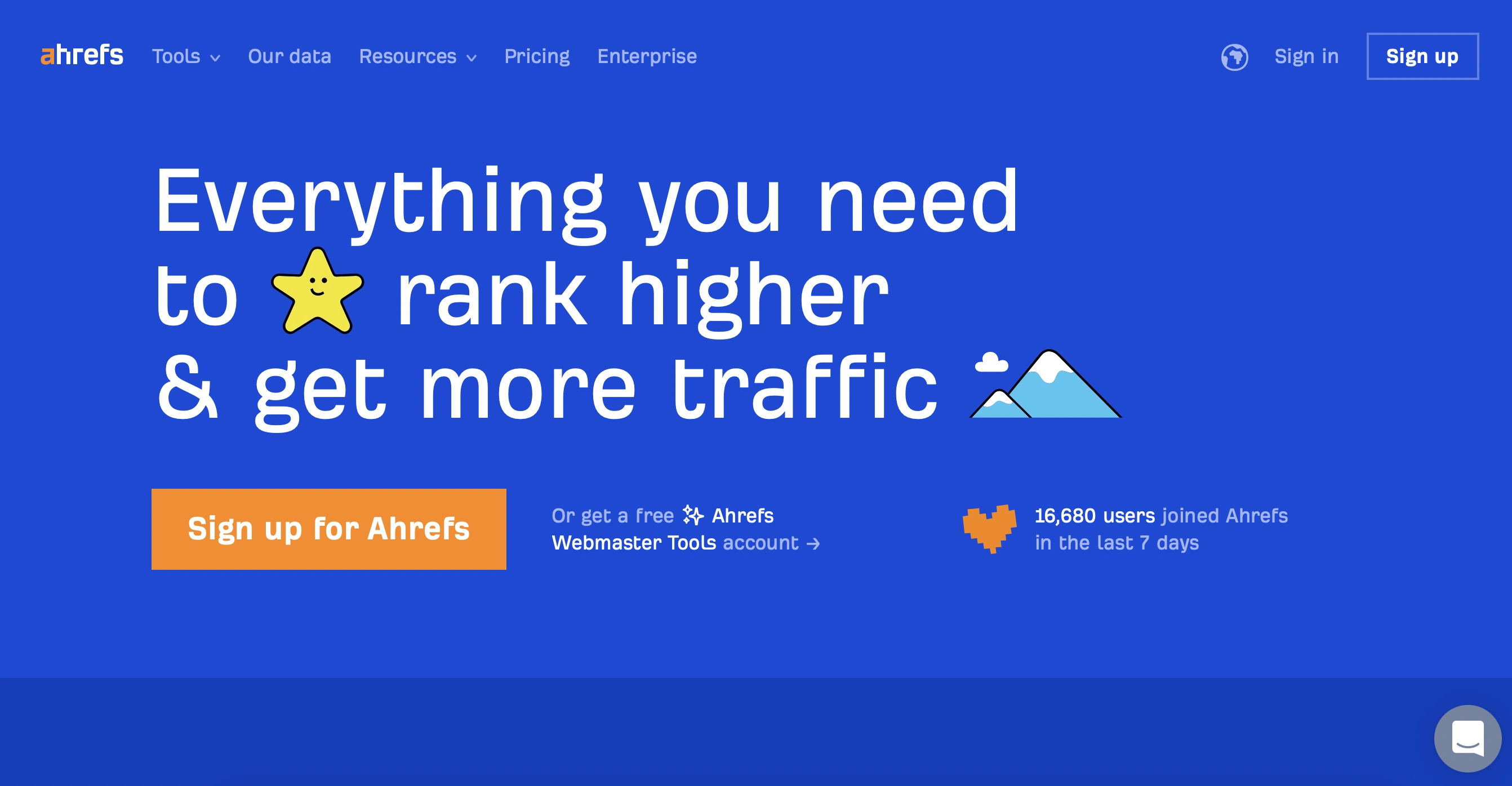This image appears to be a screenshot taken from a webpage with a visually striking and cohesive design. The background is dominated by a stunning royal blue hue, which transitions into a deeper navy royal blue strip at the bottom. At the top of the screen, the text "Ahrefs" – spelled out as A-H-R-E-F-S – is prominently displayed. Adjacent to the Ahrefs logo, there are several navigation options reading "Tools," "Our Data," "Resources," "Pricing," and "Enterprise."

On the far right of this top section, a small globe icon is visible, followed by the options to "Sign In" and a white-printed "Sign Up" button. Below this primary navigation bar, in the center of the page, a headline reads, "Everything you need to  ★ rank higher and get more traffic." Notably, the star symbol is depicted as a cheerful yellow star with eyes and a smiling face, adding a playful touch to the message.

Further down, there is a visual of a mountain capped with snow, surrounded by clouds. At the bottom of the segment, an inviting orange button labeled "Sign Up for Ahrefs" stands out, encouraging users to take action. The combined elements of color, text, and imagery create a visually appealing and informative webpage.